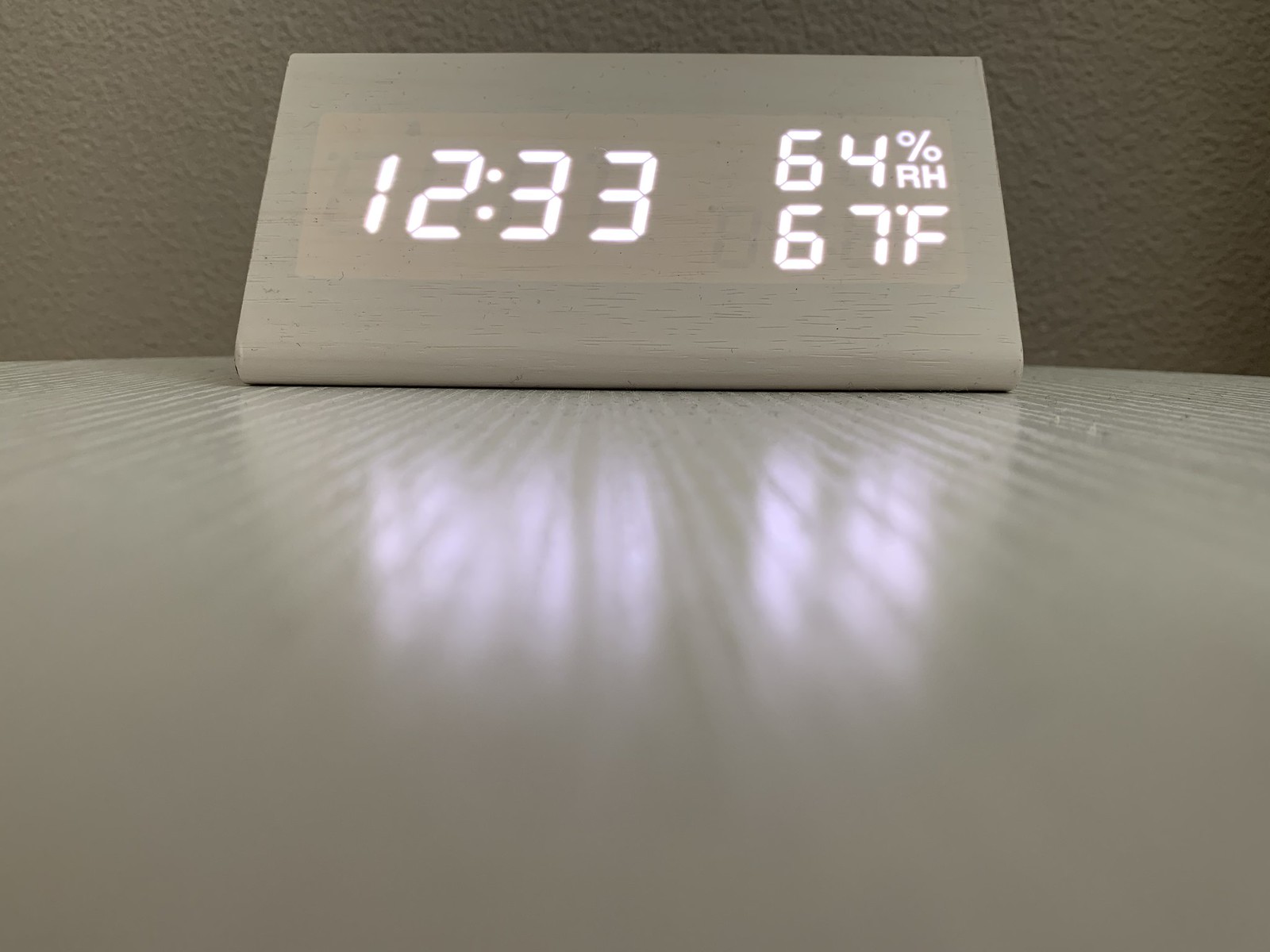This is an upward-looking photograph capturing a sleek, triangular-shaped clock resting on a smooth, white table surface. The clock has a modern design, constructed from bleached pine or white wood. It leans back into a triangular form, creating a minimalist yet striking geometric silhouette. The background wall is white, adorned with a subtle texture of tiny bumps that add depth to the scene. The pristine table surface features faint, darker lines that traverse from side to side, converging towards the center, adding to the aesthetic appeal.

The clock's face is seamlessly integrated into its rectangular front, displaying LED-style numbers and letters. The time is precisely 12:33, accompanied by the environmental readings of 64% relative humidity and a temperature of 67 degrees Fahrenheit. The clock's digital display casts a faint reflection on the glossy table, enhancing the clean and modern ambiance of the composition.